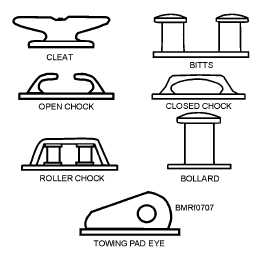The image is a detailed ink drawing of seven labeled components, each outlined in dark or black ink. 

Starting at the top left, there is a "Cleat," which is vaguely anvil-shaped. To its right, labeled "Bits," there are two cylindrical objects with caps on top. Below the cleat, labeled "Open Chock," are two hooks facing each other. Next to it, a "Closed Chock" features hooks joined at the center, resembling a bridge with an opening underneath. Further down is a "Roller Chock," depicted as two spools of thread in a container. To its right is a "Bollard," resembling a large screw without indentations. Lastly, at the bottom is a "Towing Pad Eye," drawn sideways with a hole on its right-hand side. Beside these components, there is an alphanumeric label, "BMR 10707."